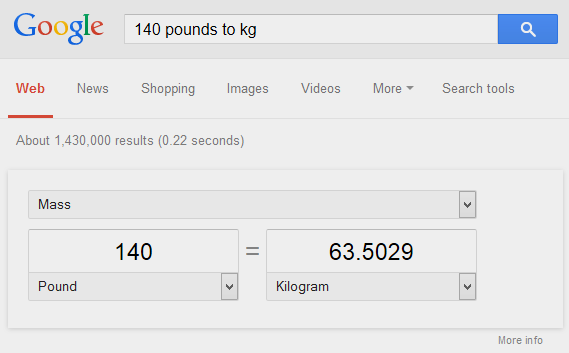The image is a screenshot of the Google search results page displayed on a desktop. Dominating the top of the page is the iconic Google logo, adorned in its traditional colors: blue, red, yellow, blue, green, and red. Immediately beneath the logo, there is a prominently placed search bar containing the query "140 lb to KG" written in black text.

Adjacent to the search bar is the familiar search icon, depicted as a white magnifying glass against a blue background. Just below the search bar, a navigation bar offers various search options, including "All," "News," "Shopping," "Images," "Videos," and "More," with "All" highlighted in red and underlined, indicating it is the current selection. The "Search tools" option is displayed in grey text.

Further down, a text line informs the user that there are approximately 1,430,000 results for the query, retrieved in 0.22 seconds, with this information rendered in grey. Below this, there is a conversion box indicating the category "Mass," featuring a dropdown arrow for further options. Directly beneath, it shows the conversion result: "140 lb is equal to 63.5029 kg," each value followed by their respective dropdown arrows.